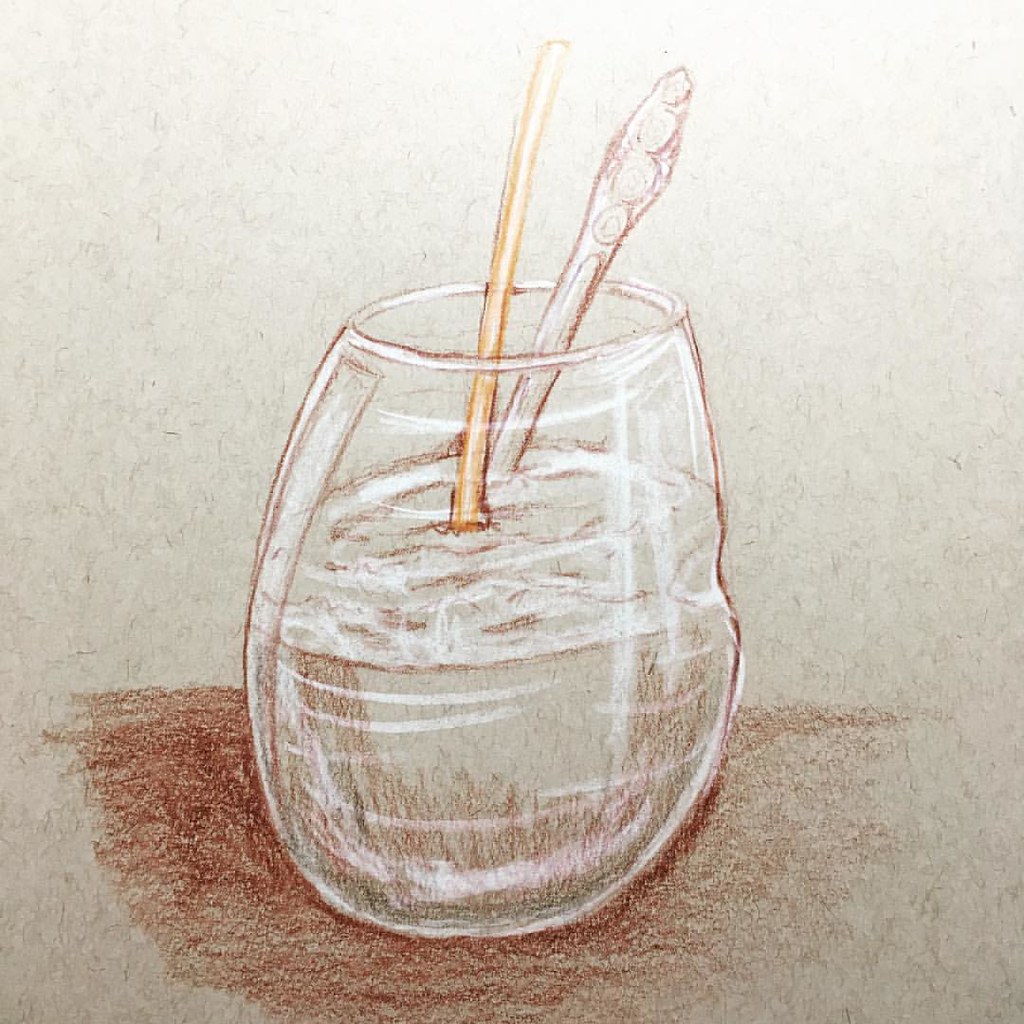This is a colored pencil drawing on a slightly mottled off-white or whitish-gray background, resembling paper. Dominating the image is a clear, stemless glass tumbler, rounded at the bottom with a slightly narrower opening at the top, giving it an egg-like shape. The glass is filled halfway with water, indicated by faint water lines, and is outlined with pink pencil marks to enhance the impression of transparency and the glass material. Emerging from the top of the glass, there's a yellow straw and a handle of a spoon, the latter adorned with three stacked circles along its edge. The handle protrudes ambiguously, conjuring thoughts of a possible toothbrush due to its design. Beneath the glass, there's a shaded, semicircular area rendered in a brownish-red tone, giving the appearance of a shadow and suggesting the glass is seated on a table.